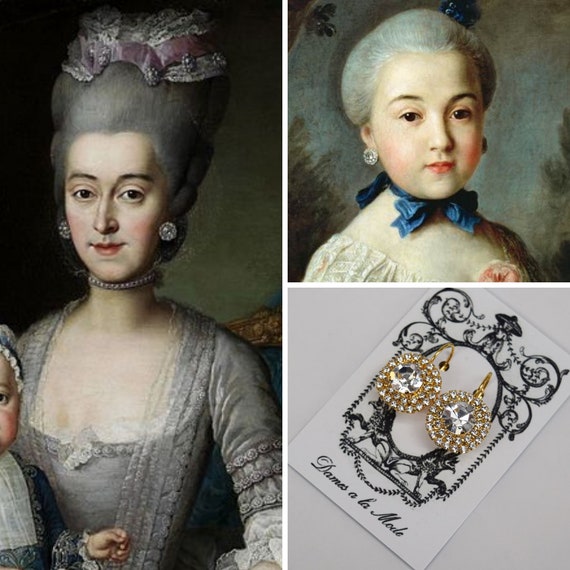The collage consists of three images. Dominating the left 50% is a tall, Victorian-era painting of a woman with tall, gray hair styled in a beehive with a hair ornament shaped like an upside-down 'U' adorned with white lace. Her appearance is almost ghostly, with dark eyebrows, dark eyes, and she wears prominent diamond earrings that add an air of opulence. She is dressed in a gray bodice dress with white lace detailing and a high pearl choker necklace. A child in a blue, lace-edged outfit sits on her lap, adding a maternal aspect to the scene. 

On the right side, divided into two equal sections, the top half features a portrait of a young girl with chubby cheeks and white or grayish hair tied in a blue ribbon around her neck. She also dons the same distinctive large diamond earrings and has black eyes and dark eyebrows, echoing the mysterious elegance of the woman on the left. 

The bottom right image showcases these diamond earrings again, displayed on a card with cursive text that reads "Dames a la Mode," emphasizing a historical or fashion context. The shared elements of the lace dresses, the striking earrings, and the detailed adornments create a cohesive and haunting visual narrative between the images.